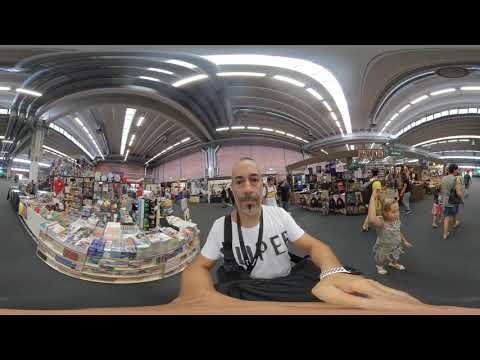The image features a fisheye distortion that bends and curves the scene dramatically. At the center stands a middle-aged white man with a gray beard and mustache, thin balding hair, and a white shirt featuring black letters, including a visible "P" and "E." He is holding a 360-degree camera, with its black lanyard hanging around his neck, and the lower part of his arms and hands appear exaggerated and distorted due to the lens effect. He wears a wristwatch on his left wrist.

In the background to the right, a small blonde child raises her right arm, and various people are seen walking away with their backs to the viewer. The setting appears to be indoors, possibly in a convention center or shopping area, with curved ceilings lined with a long bank of lights. The surroundings include multiple market areas and shops displaying an assortment of items and packaging. Large metal girders support the ceiling, and the floor is covered in gray carpeting. The scene is filled with vibrant colors, including black, white, gray, green, blue, red, orange, light green, and tan.